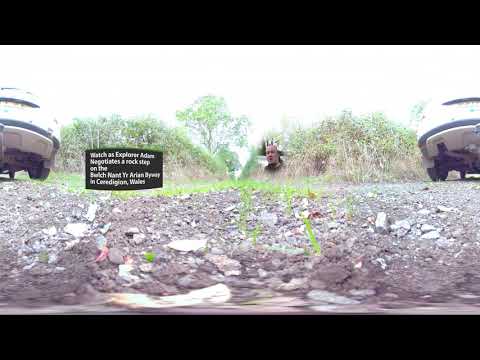This image captures a rugged outdoor scene. It features a rocky, dirt-strewn field in the foreground, dotted with patches of grass. Two trailers or boats flank the left and right edges of the image, partially visible. In the background are two similar-looking hills, with a single tree atop the one on the left. The sky is overcast, painted in shades of gray and white. Amid the foliage, a man in his 40s, presumably "Explorer Adam," is visible. At the top and bottom of the small, rectangular horizontal image are thick black bars. Text appears on a black rectangle positioned in front of the left hill, written in white letters and partially readable, stating, "Watch as Explorer Adam negotiates a rock step on the… in… whales." The colors in the image span a natural palette of browns, grays, whites, greens, and other earthy tones, suggesting an advertisement, perhaps for a YouTube channel.